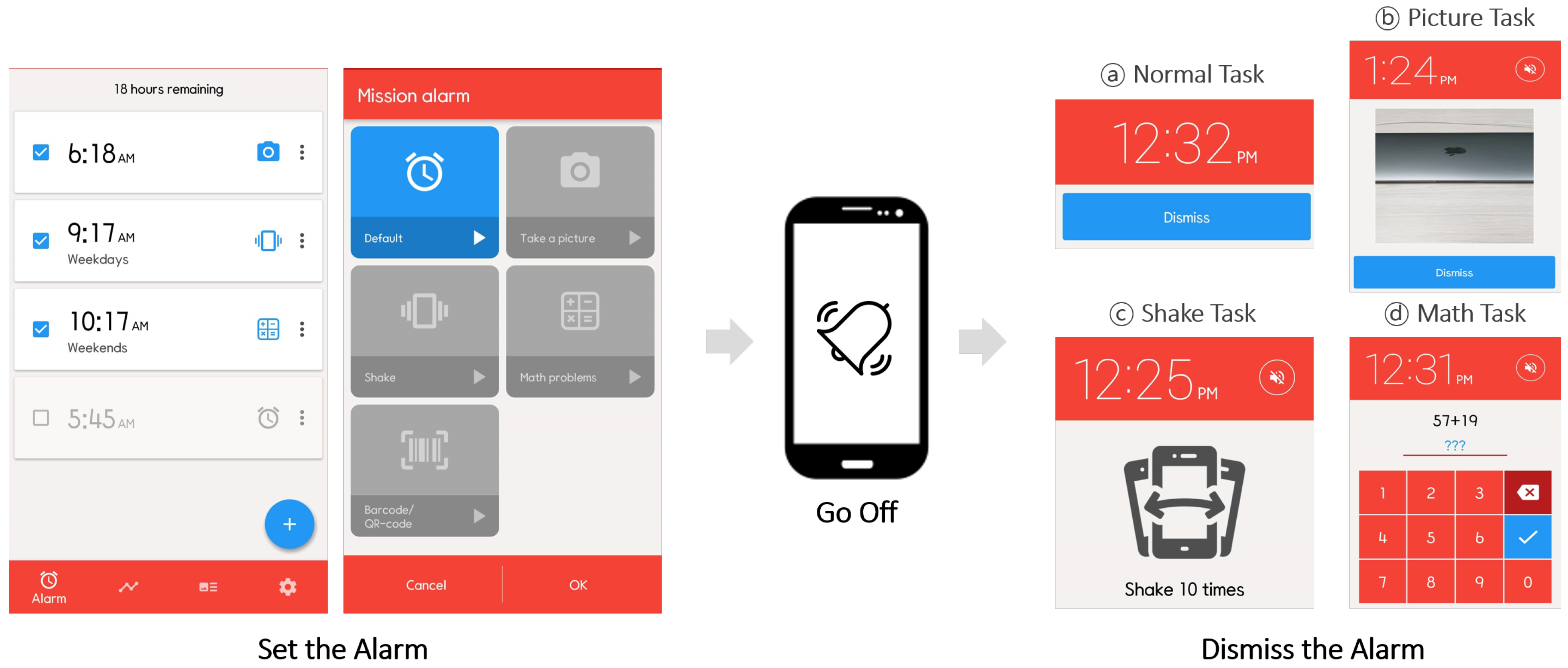The image is a detailed illustration of an alarm app interface on a cell phone, demonstrating various functionalities and tasks required to dismiss an alarm. Occupying the central position is the phone with a white screen encased in black, featuring a bell icon and the text "go off" in the center. On the left side of the phone, there is a box displaying "18 hours remaining" along with three set alarm times: 6:18, 9:17, and 10:17, each marked with a blue check to indicate they are active. Further right, the interface includes red text reading "mission alarm" alongside options, including "default," "take a picture," "shake," "math problems," and "barcode QR code" in gray text. 

To the right of the phone, another section outlines tasks labeled "normal task" and underneath shows the current time, "12:32 p.m." Below this, there are three tasks: a shake task, a picture task, and a math task, each accompanied by a blue "dismiss" button. Specifically, the math task includes a red calculator icon with white numbers. This setup illustrates the app's diverse methods for alarm dismissal, whether by shaking the phone, solving math problems, or taking a picture.